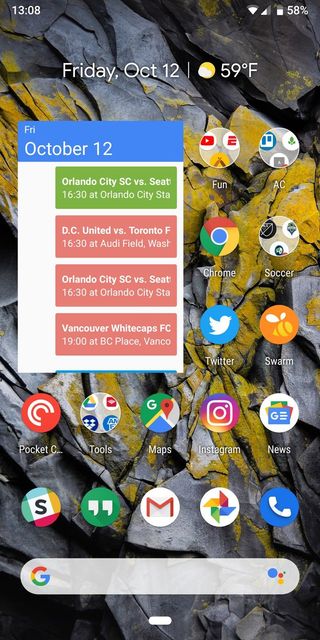This is a detailed screenshot of someone's cell phone home screen. At the very top of the screen, the status bar displays the time as 13:08, with a battery life of 58%. It is Friday, October 12th, and the weather is 59 degrees Fahrenheit, indicated by an icon of a sun partially obscured by a cloud. 

Below the status bar, the screen displays a series of events for the day, specifically soccer matches:
- **Friday, October 12th:**
  - Orlando City SC versus Seattle at 16:30 at Orlando City
  - D.C. United versus Toronto at 16:30 at Audi Field, Washington
  - Orlando City SC versus Seattle at 16:30 at Orlando City Stadium (presumably a repeated mention)
  - Vancouver Whitecaps at 19:00 at BC Place, Vancouver

There is a grid of app icons prominently displayed on the home screen. The apps include:
- Fun
- AC
- Chrome
- Soccer
- Twitter
- Swarm
- Pocket
- Tools
- Maps
- Instagram
- News

There are also a few unlabeled icons:
- One icon with an 'S' in the center.
- A green icon with white quotation marks in the center.
- An icon for Google Mail (Gmail).
- A multi-colored pinwheel icon representing Google Photos.
- A blue icon featuring a white telephone handset for the Phone app.

At the very bottom of the screen, there is a Google search bar, currently empty. The image orientation is portrait, being taller than it is wide.